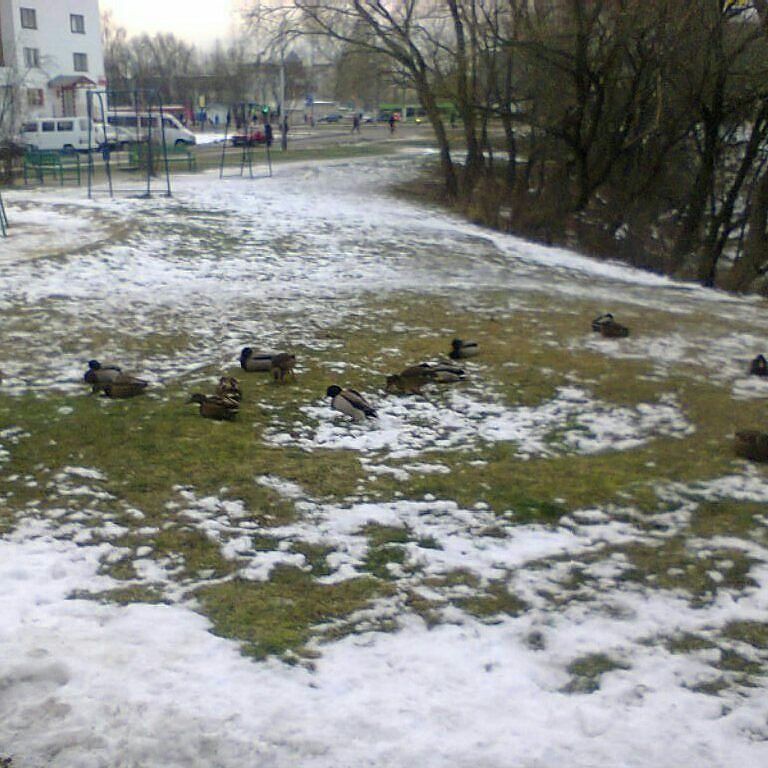The image is a square, color photograph taken outdoors during the daytime, depicting a snowy park scene. Snow partially covers the ground, revealing patches of dark green, light yellow, and brown grass in the center. In the foreground, a small flock of about ten ducks, characterized by their brown feathers and darker heads, are scattered around; some are sitting while others walk and peck at the ground. In the background to the left, near the edge of the grassy patch, there is a playground area featuring green metal-framed swings and several benches positioned behind them. A white, multi-storeyed building with six visible windows and what appears to be white minivans are situated further in the distance, adjacent to a road. On the right-hand side of the image, there are mostly bare, dark-limbed trees with some brown leaves clinging to the branches. The very distant background reveals the grainy, blurry silhouettes of people walking, their legs splayed apart, and the outlines of larger, obscured buildings.